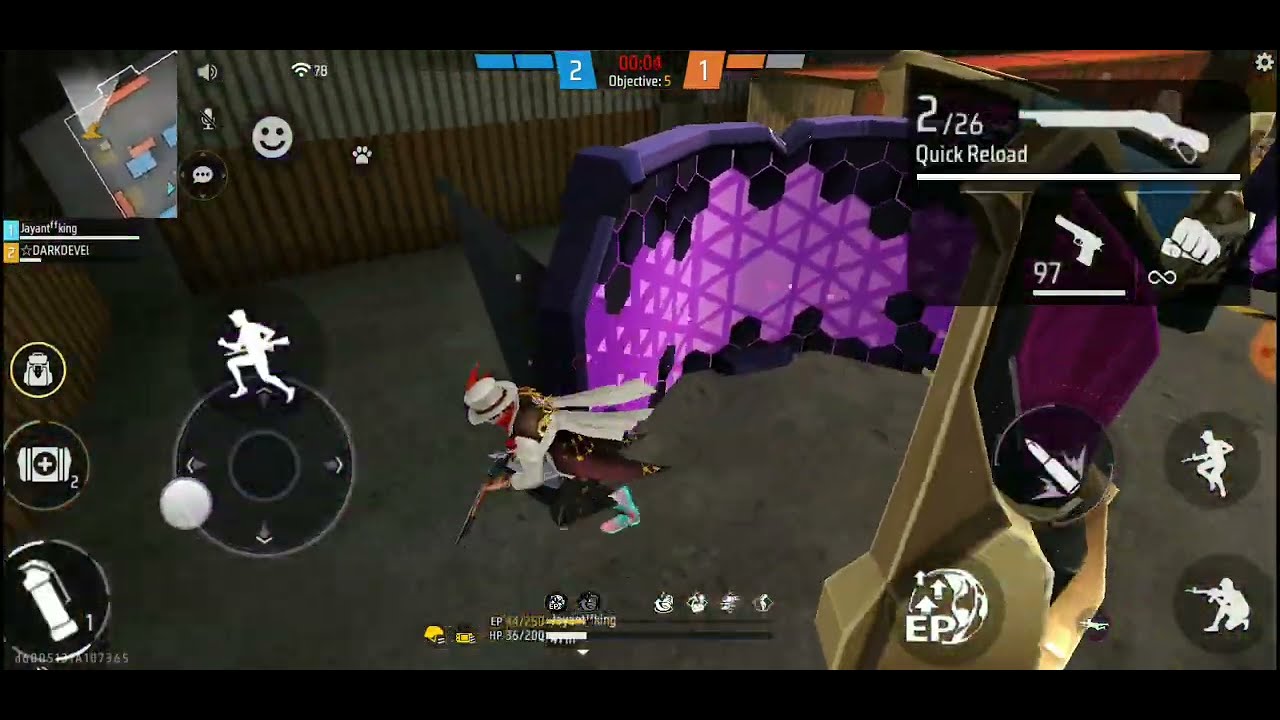The screenshot captures an intense moment in a mobile shooting game. Dominating the screen is a character in the middle, resembling a cowboy, wearing a white top hat, a long trench coat, and striking blue and purple boots. The character holds a large shotgun and stands against a backdrop comprising gray concrete flooring and brown corrugated metal walls. 

To the top right, game statistics are displayed: "2/26" next to an image of an old-school rifle, "97" next to an animated image of a handgun, and an infinity symbol below a fist image. "Quick Reload" is indicated near these weapon icons. A happy face icon is visible on the left side, contributing to the in-game HUD details. 

Additionally, a mini-map is located at the top left corner. The left-hand side of the screen displays controls including a joystick, a grenade button, and icons for med kits and backpacks. On the right, action buttons such as 'fire,' 'crouch,' and 'stand' surround an icon of a world globe with "EP" and three arrows on top. The setting is partially defined by purple barriers with a honeycomb pattern, suggesting a factory-like environment. 

In the bottom left corner, two soldier outlines in combat stances add to the scene's tension—one standing with a gun, the other crouching. Overall, the intricate overlay of controls, weapon stats, and strategic elements paints a comprehensive picture of the gaming experience.